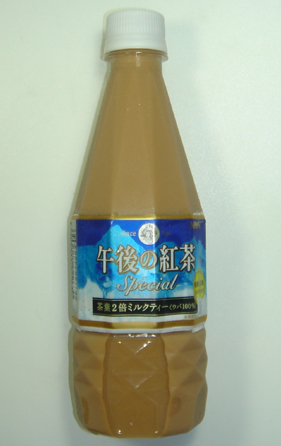This close-up photograph showcases a plastic bottle with a white twist cap lying on a white surface. The bottle contains a caramel brown or tan-colored liquid. Its cylindrical shape widens at the bottom and tapers toward the top, featuring ribbing for grip near the base. The label, predominantly blue with a picturesque mountain scene—dark blue at the top transitioning to white at the bottom, suggestive of a snow-capped range—is adorned with Chinese writing. Additionally, there is some Japanese text towards the bottom, along with an English word "special" positioned between the Asian characters. The label also includes a gold circular seal with more text. The bottle's setting against a white background adds to the simplicity of the image, highlighting the detailed design and vibrant colors of the label. Despite the liquid's vague appearance, it strongly resembles a caramel or malt beverage.